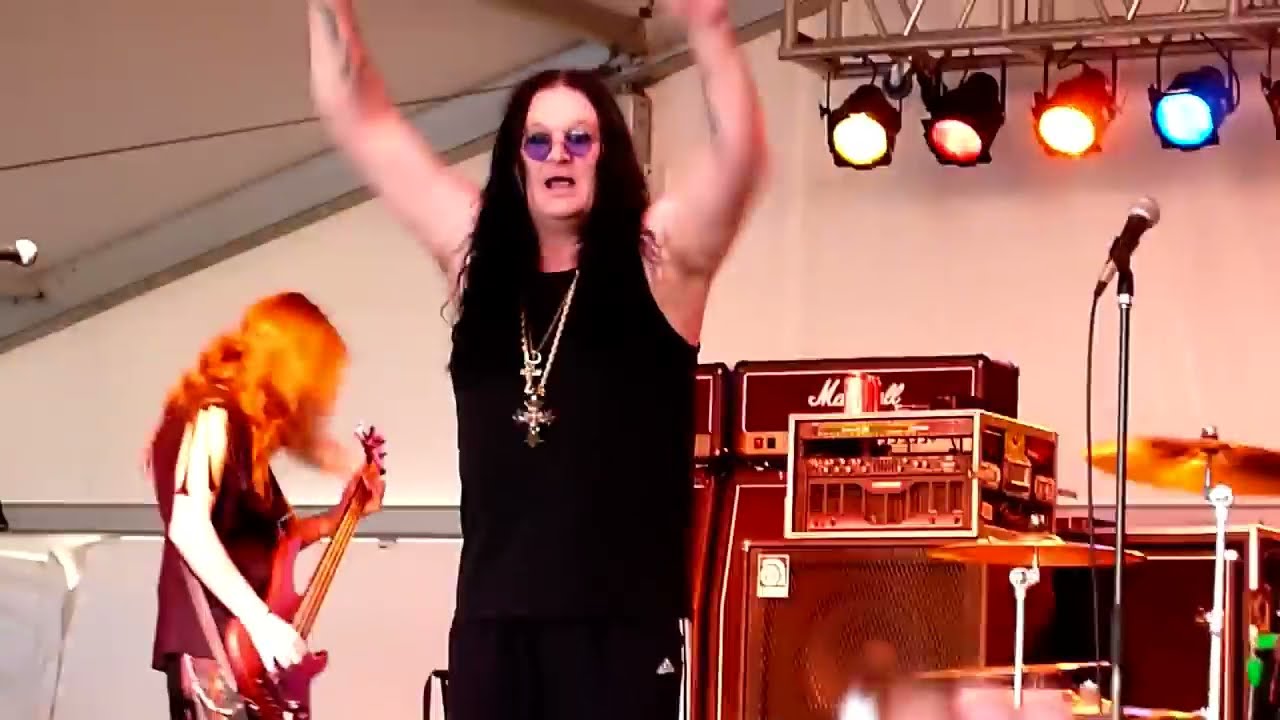The image captures a dynamic performance scene featuring a visibly aged Ozzy Osbourne. He is standing just left of center, wearing a sleeveless black muscle shirt and what appear to be black Adidas shorts or sweatpants with a vertical white stripe. His long, black hair cascades down to his shoulders, and he is adorned with numerous pieces of jewelry, including several golden chains, at least two crosses, and a ring attached to one of the necklaces. Ozzy's arms are raised above his head, blurred in motion, and his mouth is open, suggesting he is singing or shouting. He sports circular, purple-tinted sunglasses. 

In the background and slightly to the left, a bassist with long, flowing red hair, obscures their face with their locks. It is likely that the bassist is female, judging by the musculature of the visible arm. She is playing a red guitar and is also dressed in a black tank top. The stage setup includes various equipment: Marshall amplifiers, speaker stacks, a black microphone on a silver stand, and several drum cymbals towards the bottom right. Overhead, a bank of multicolored stage lights illuminates the scene, suggesting this performance is taking place under a large white tent. The overall ambiance is energized by the visible motion and vibrancy of the stage setup.